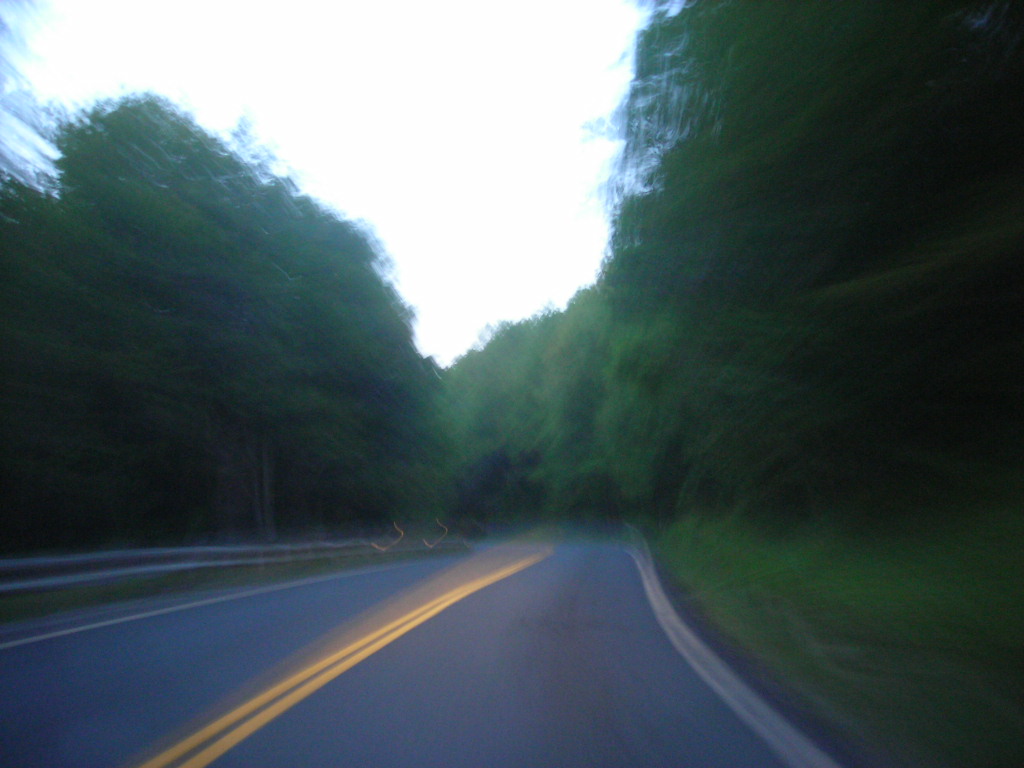A photograph taken from the perspective of someone inside a car, looking down a deserted, dark gray tar-covered road that winds through a heavily wooded countryside. The road features a double yellow line running down its center, with a faint lighter white or off-white edge line on both sides. On the left-hand side, just past the edge line, there's a steel silver guardrail running parallel to the road. This side of the image is dominated by a high line of dark green trees that continue all the way from the bottom to the top of the image. The far end of the road curves off to the left, disappearing into a thick tree line that spans across the background. On the right-hand side of the road, a white line edges the pavement, and above the line is a stretch of green grass leading up to more dense trees. The sky above is a bright white, indicating daytime, possibly with the sun shining brightly. The image is somewhat blurry, giving the road markings a smudged appearance and emphasizing the thick, encompassing greenery of the tree-lined road.